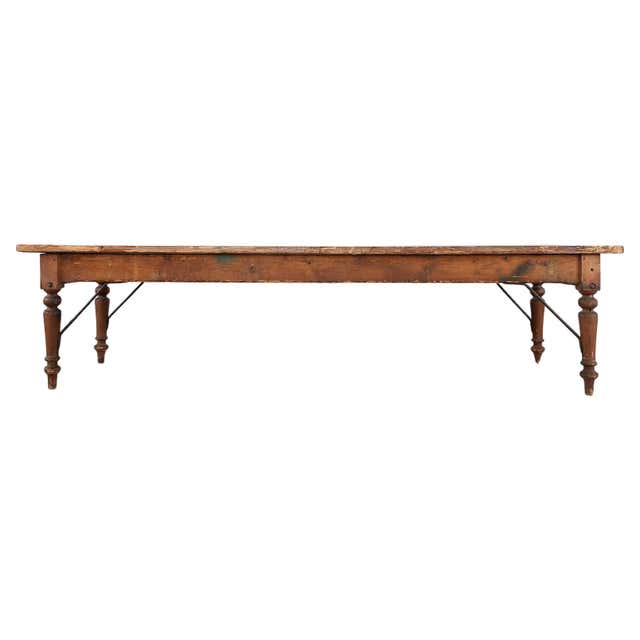This image showcases a long, vintage wooden table, viewed from the side against a white background for a product photo. The rectangular table exhibits signs of wear and age, including black marks throughout its surface, suggesting it is an older piece, possibly an antique. The table features four stubby legs, each with a distinctive design: a ball at the top followed by a rod-like section that extends to the ground. Additionally, small rods are attached from the legs to the table, likely for added stability. The overall appearance of the table conveys sturdiness and gives the impression of a coffee table, reminiscent of accent pieces you'd find in an antique shop or a grandparent's home. This table is presented as an item for sale.